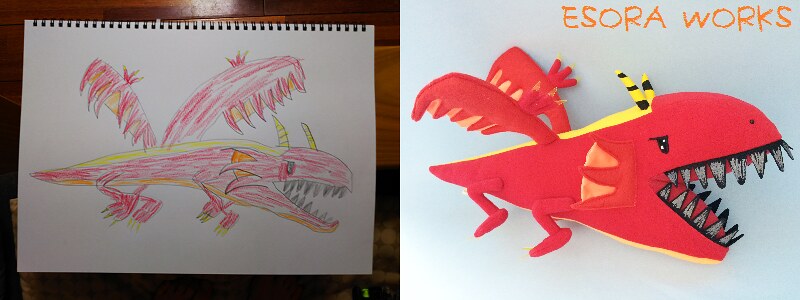This is a composite image featuring two artworks displayed side by side. The right side showcases a vibrant illustration or painting of a fantastical, mythological creature with a red whale-like body, equipped with large, red wings on top. The creature is uniquely hybridized with two human-like legs in place of traditional fins. It faces rightward, baring grey teeth and a grey eye, and is adorned with two antler-like or antennae structures in red and black. Additionally, it boasts a subtle yellow and black accent on its back. The artwork is set against a grey background, with the text "Asura Works" inscribed in orange at the top.

On the left side, the image presents a pencil drawing of a similar creature on white paper, held in place by a binder clip at the top. This sketch is laid on a wooden surface. The penciled beast shares resemblance to its colored counterpart but is rendered with four legs instead of two. The antlers are depicted larger, and the wings, detailed with tooth-like structures on the right side, add to its fantastical nature. The top of this sketched creature is shaded in yellow, offering a hint of color amidst the otherwise monochromatic artwork.